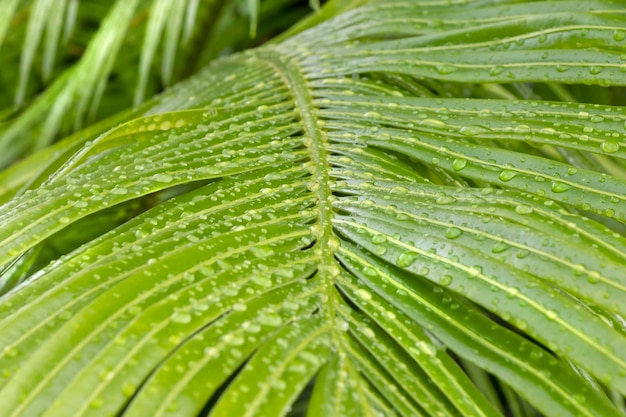This image is a close-up, macro shot of a vibrant green leaf, likely from a tropical plant such as a fern or palm, accentuated by the recent rainfall. The leaf, bent and adorned with droplets of water, showcases a rich spectrum of green hues that convey a sense of freshness and vitality. Thin but prominent veins, including a central main vein, traverse the leaf, adding delicate yellowish patterns. The surface of the leaf has a waxy texture, further emphasized by the glistening raindrops dispersed across it. The background consists of additional green foliage, slightly out of focus, ensuring the central leaf remains the focal point of this rainforest-like scene.